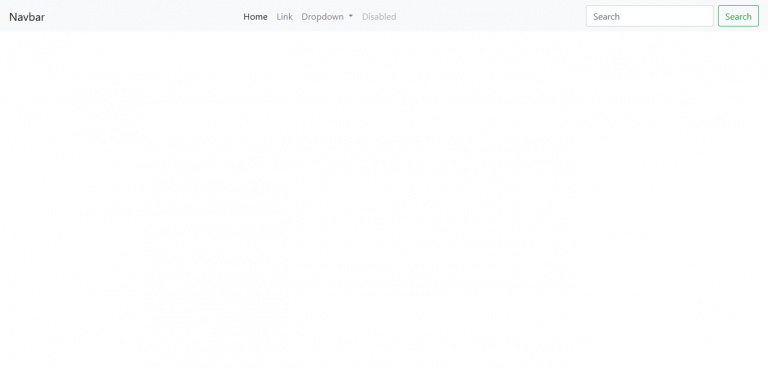Caption:

The image showcases the top section of a computer screen featuring a minimalistic menu bar. The menu bar is displayed in gray and contains various elements. On the left, the label "NAVBAR" is prominently displayed in capital letters, hinting that this could either be a navigation component or possibly the name of a company. Centered on the bar are four menu options: "Home," "Link," "Dropdown," and "Disabled." The "Home" option is distinctly highlighted, indicating the current selection, while the other options appear grayed out, suggesting they may not be interactive. On the right side of the menu bar, there is a search box accompanied by a green-highlighted search button. The overall interface is simple, and the limited context makes it challenging to infer the specific application or purpose of this menu bar.